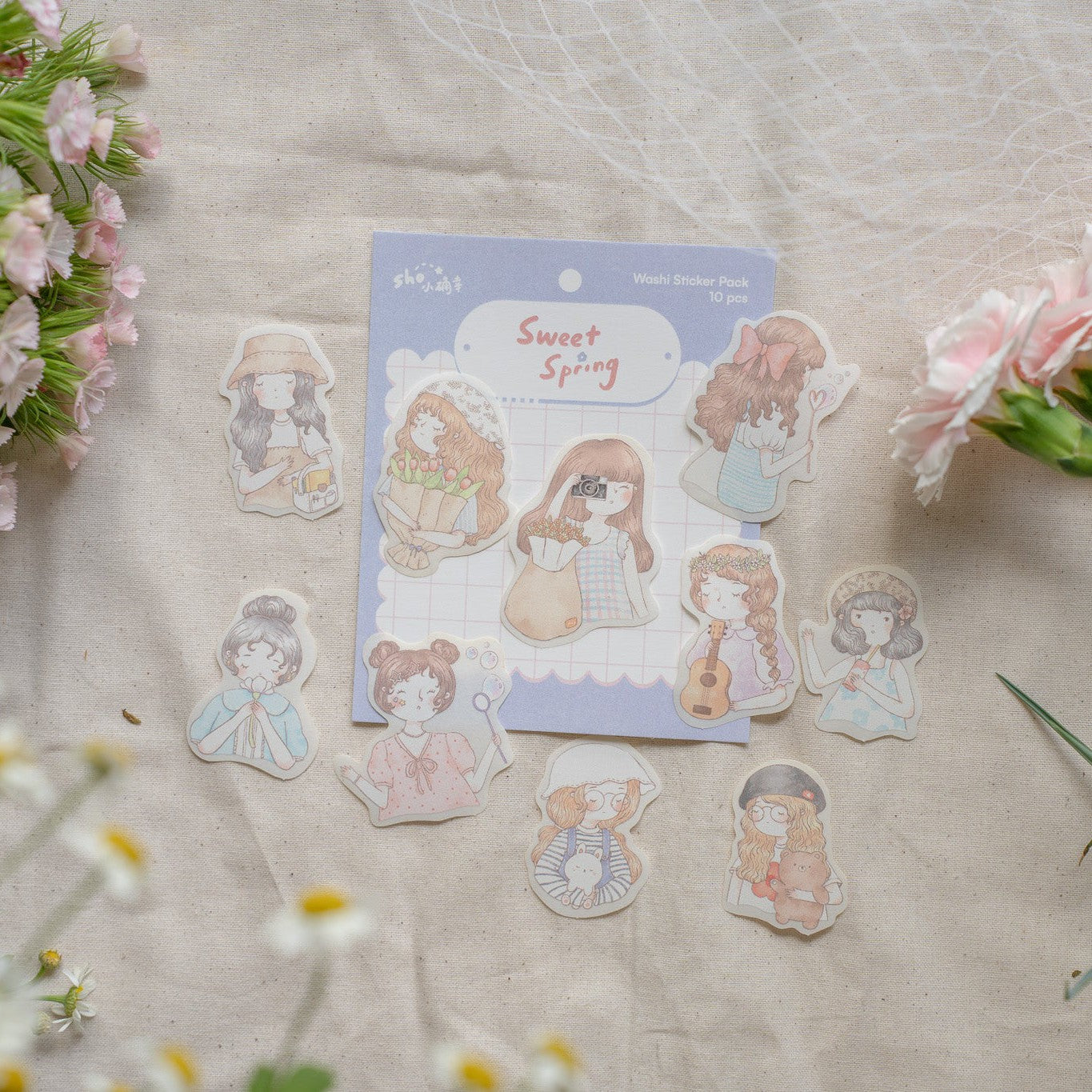The image features a detailed sticker pack titled "Sweet Spring" displayed on a white surface adorned with pink carnations and daisies. The pack consists of 10 stickers, each depicting a cartoon girl with brown hair. One sticker shows a girl with a camera, capturing a moment, while another depicts a girl hugging a sack of flowers. A different girl is shown holding a guitar, and another appears with a pencil topped by a heart-shaped eraser. All figures are engaged in various activities, mostly flower-related, creating a cohesive and delightful spring-themed collection.